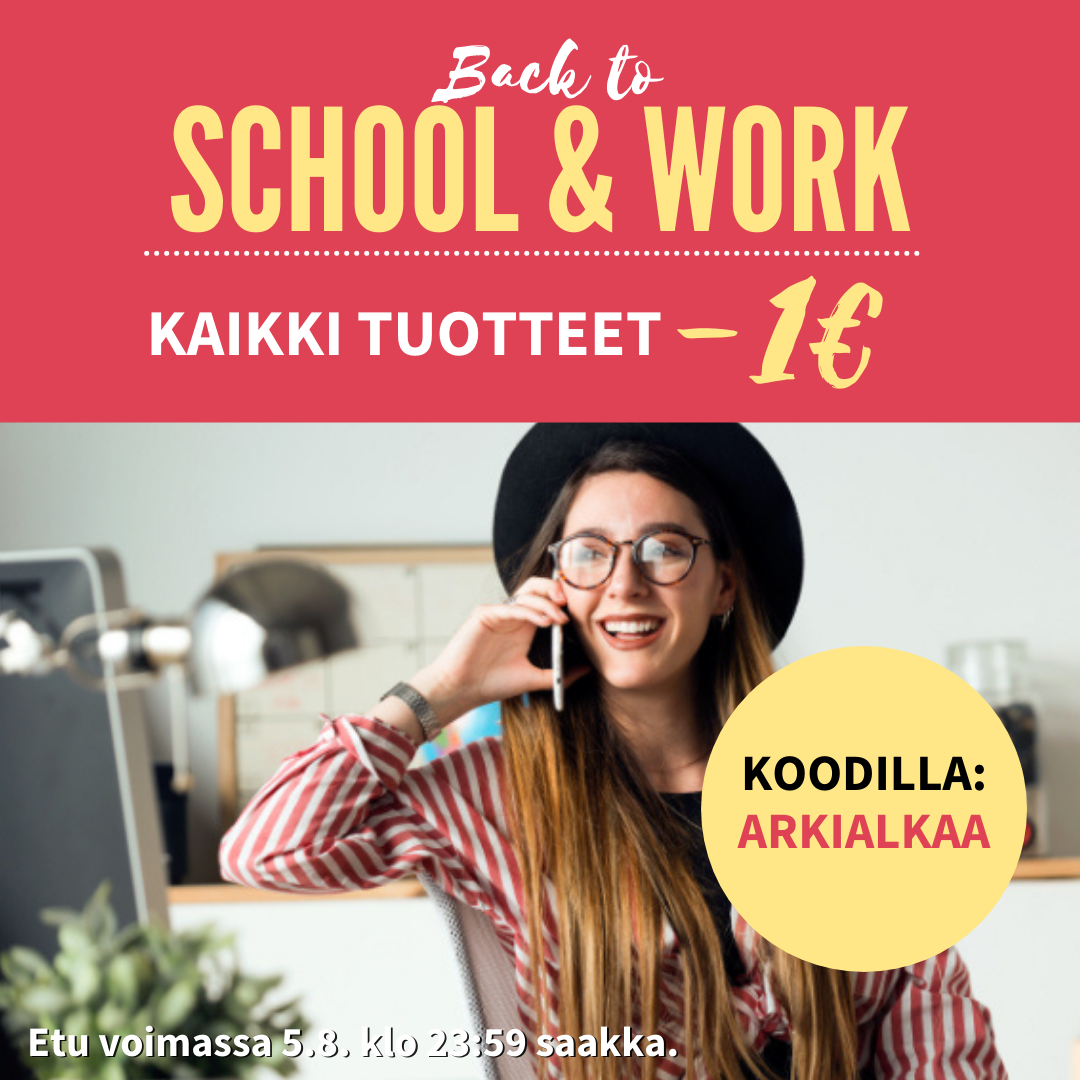The advertisement features a prominent red rectangle at the top with the headline "BACK TO SCHOOL AND WORK." The words "Back to" are written in a white cursive font, while "SCHOOL AND WORK" are in all-caps yellow letters in a more serious, larger font. Below this headline, there's a dotted line with white typography spelling out "KAIKKI TUOTTEET," followed by a yellow dash and the symbol "1€."

The central part of the image showcases a cheerful woman talking on her cell phone. She is dressed in a red and white vertical striped shirt and a black hat, accessorized with a silver watch on her right hand and eyeglasses. She has long brown hair with highlights and is smiling broadly, revealing her white teeth adorned with red lipstick. The background gives an impression of an office setting, featuring a blurred gray desk lamp and a plant in the bottom left-hand corner.

Additional text elements are present, including a yellow callout with the text "Kudila Arkealka," and some more information in the bottom left corner that reads, "et tu, Vuamasa? 5.8 KLO 2359 Saco." Overall, the image seems to advertise a service or product for back-to-school and work, with details and pricing indicated in another language.